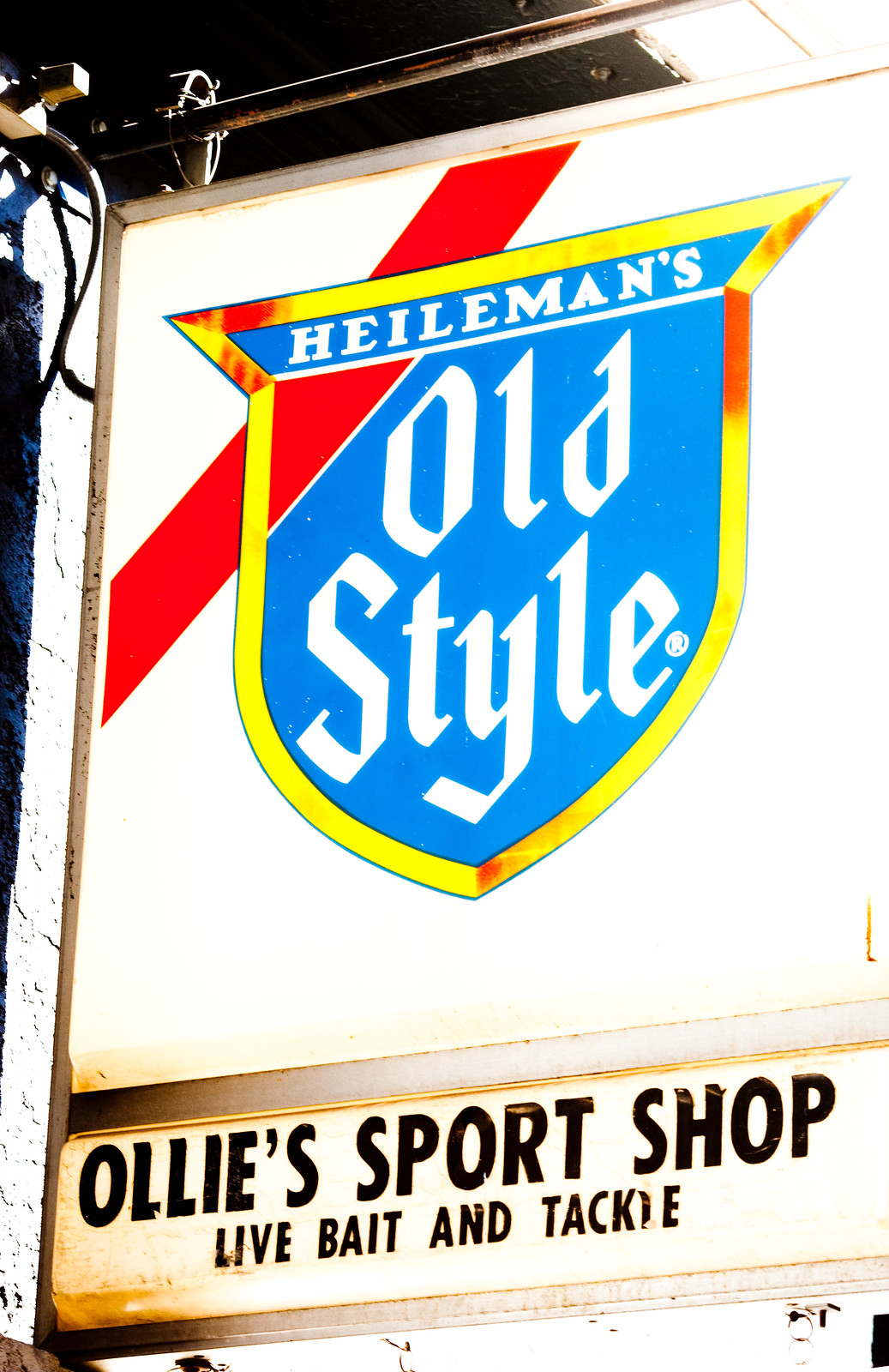The close-up image shows an aged, illuminated sign hanging from a pole outside a building, taking up the entirety of the frame. The sign is divided into two sections on a white background, with visible yellowing likely due to weathering or internal light burn. The upper, larger section displays a logo for "Heileman's Old Style," a type of beer, designed on a gold shield with a red diagonal stripe. The shield has a blue background with white text: "Heileman's" at the top and "Old Style" below. The red stripe on the shield continues into the white background of the upper sign section. Below, the smaller rectangular section features "Ollie's Sports Shop Live Bait and Tackle" in plain black text, with no additional logos or branding. The image captures both sections clearly, alongside a glimpse of the adjacent brick building.